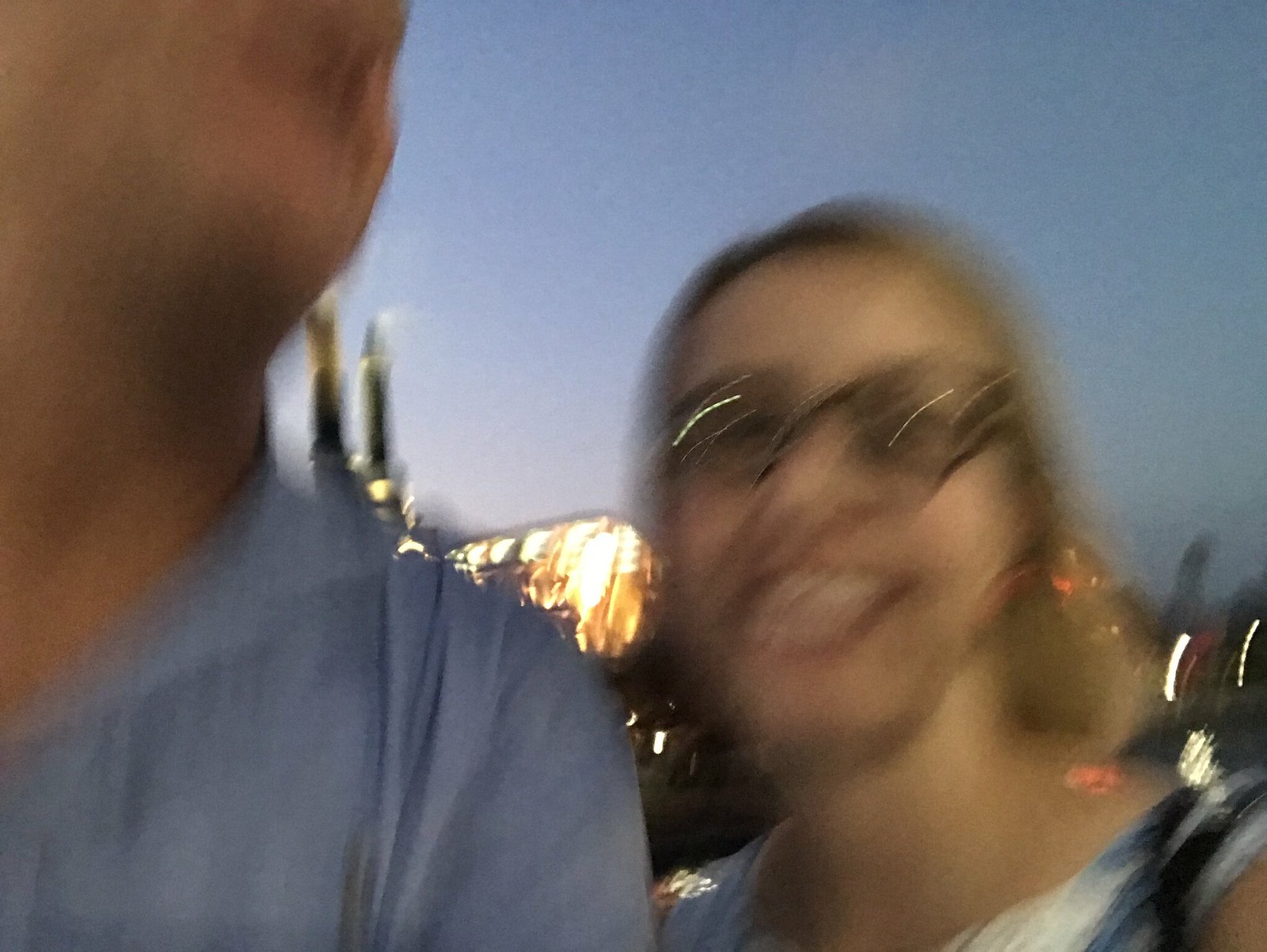Against a deep, midnight blue backdrop, a bright, white light—reminiscent of an LED or light bulb—illuminates the scene, casting a radiant glow. On the right side of the image, a person with a radiant smile poses for the camera. Although the shot is somewhat blurry, you can distinguish their black glasses and the vibrant lipstick they are wearing. Their attire consists of white and blue, adding a crisp contrast to the blue tones of the background. Another person is faintly visible beside them, but their face is entirely indiscernible due to the graininess of the image. They are dressed in a light blue, slightly wrinkled shirt. The overall image has a grainy texture, adding a nostalgic or retro feel to the composition.